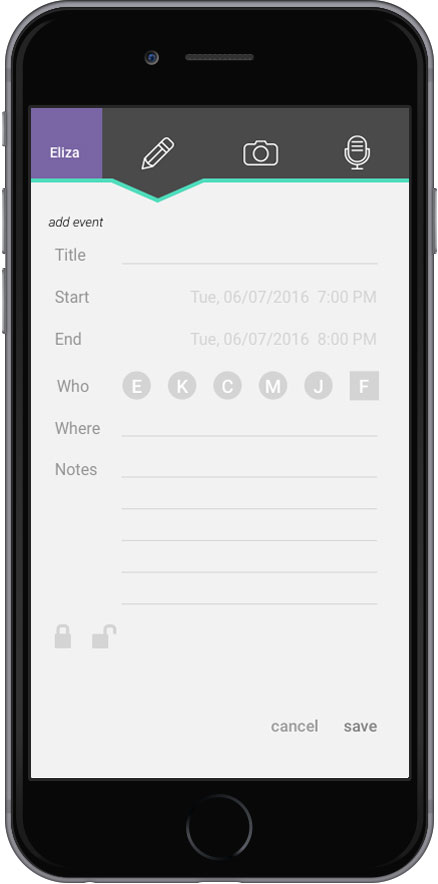The vertical image showcases a black smartphone positioned against a white computer screen background. The phone, likely encased in a design with a light gray strip along its edges, features visible side buttons including the power button, volume controls, and other switches. The camera is located at the top of the device.

The screen displays the smartphone's homepage. On the upper left, a purple square with the white text "Eliza" stands out. Adjacent to it, a dark gray section includes icons resembling a pencil, camera, and microphone. The remaining screen space displays a predominantly white background with several text sections and icons.

In detailed view, the text "Add Event Title" appears in gray or black, followed by lines for input. Below, event details read: "Start Tuesday, 6-07-2016, at 7 p.m." and "End Tuesday, 6-07-2016, at 8 p.m.," both in a faded gray color. Further down, there is a section labeled "Who," accompanied by circles containing the initials E, K, C, M, J, and F, alongside another input line. The "Notes" section features multiple lines for text, though none are filled in.

At the bottom of the screen, a padlock icon is displayed in an unlocked state, and the "Cancel" and "Save" buttons are visible in the bottom right corner. Additionally, the smartphone's physical home button is located at the very bottom of the device.